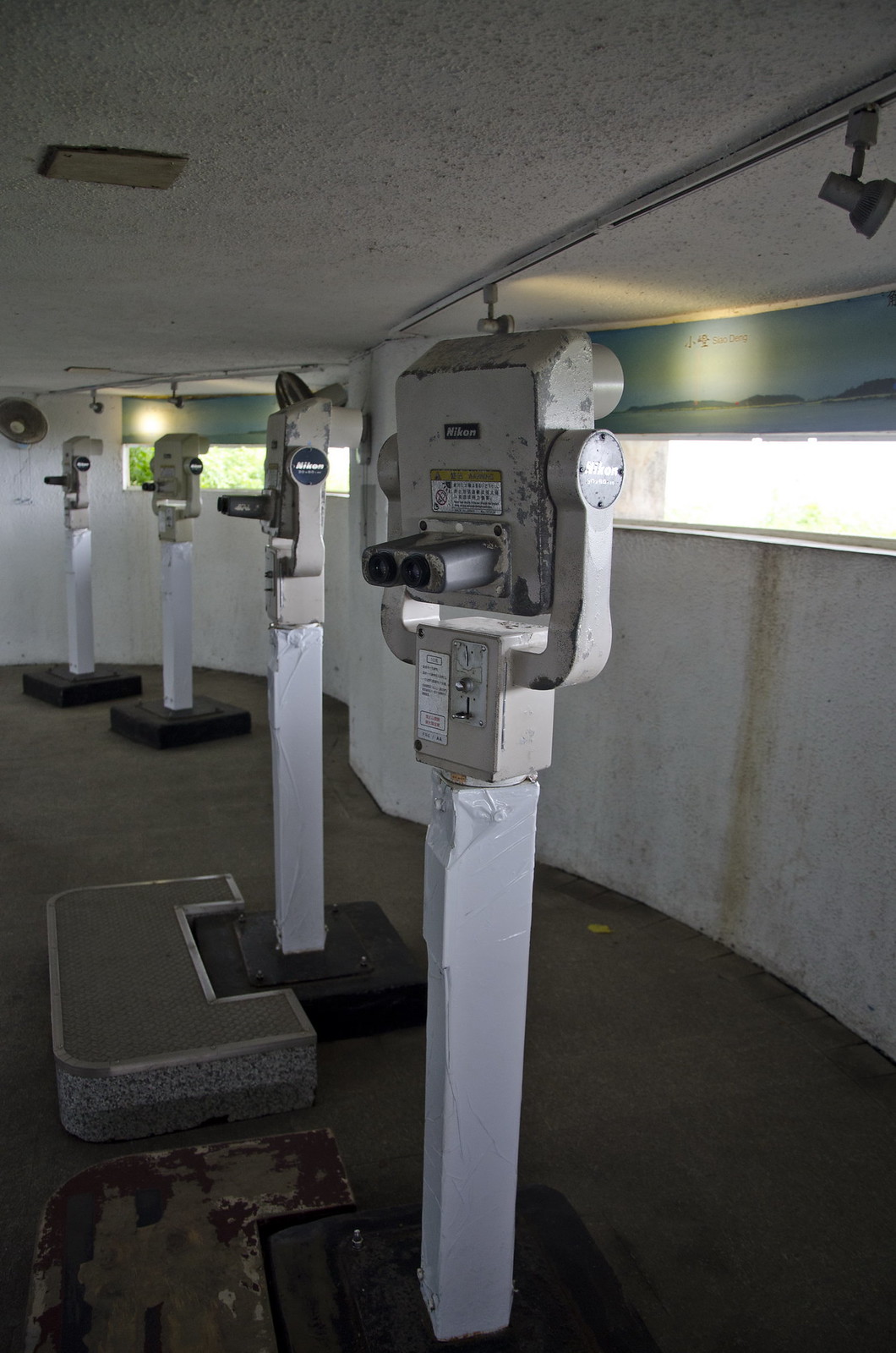The photograph depicts a concrete room with a thin, horizontal window running along the length of one wall, casting light into the otherwise enclosed space. The room houses four mounted viewfinders designed for improved viewing experiences often found at lookout points or historical monuments. Each device rests on a white pole anchored to the ground by black square bases. The viewfinders themselves are primarily white, accented by black eye holes for viewing. Two of the viewfinders are accompanied by a small stool, enabling shorter individuals to comfortably look out through the lenses. The room's austere aesthetic is defined by its concrete floor and walls, providing a stark backdrop to the precision and utility of the viewfinders.